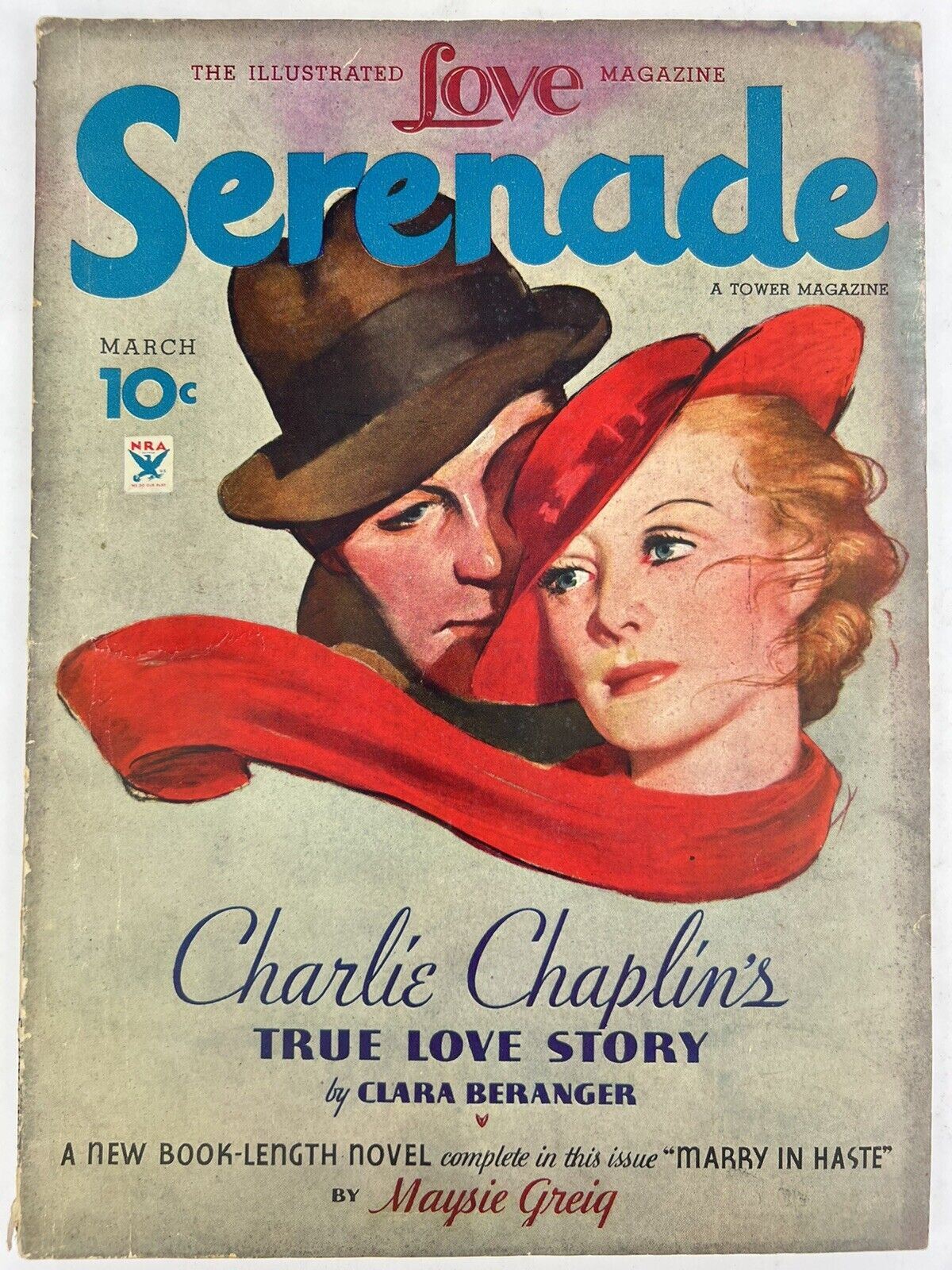This vintage magazine advertisement, printed on beige paper with slightly torn edges, captures an old-fashioned allure reminiscent of the 1920s to 1940s era. At the top, in bold red capital letters, it announces "The Illustrated Love Magazine," with "Love" in a larger font. Below, "Serenade" is prominently displayed in large blue letters, followed by the phrase "A Tower Magazine" in smaller black capitals to the right. The issue is from March and is priced at Ten Cents, denoted in blue below the heading, with an NRA stamp situated below it.

The centerpiece of the cover features a painted image of a man and a woman. The man, wearing a brown top hat, is partially visible, with only his right eye and nose fully shown as his face is partly obscured by the woman. The woman, adorned with a red hat tipped to her right (viewer's left) and a flowing red scarf around her neck, turns towards the left, revealing her red hair, thin eyebrows, blue eyes, and pink lipstick. Both individuals are depicted as white.

Beneath this illustration, the caption "Charlie Chaplin's" appears in dark blue cursive, followed by "True Love Story" in bold blue capital letters, and "by Clara Beranger" in thinner blue writing. Further down, in black text, the cover promotes a new book-length novel complete in this issue, "Mary in Haste" by Maisie Greig, with Greig’s name highlighted in red. The entire background maintains a matted sepia tone, enhancing the nostalgic feel of this classic magazine cover.